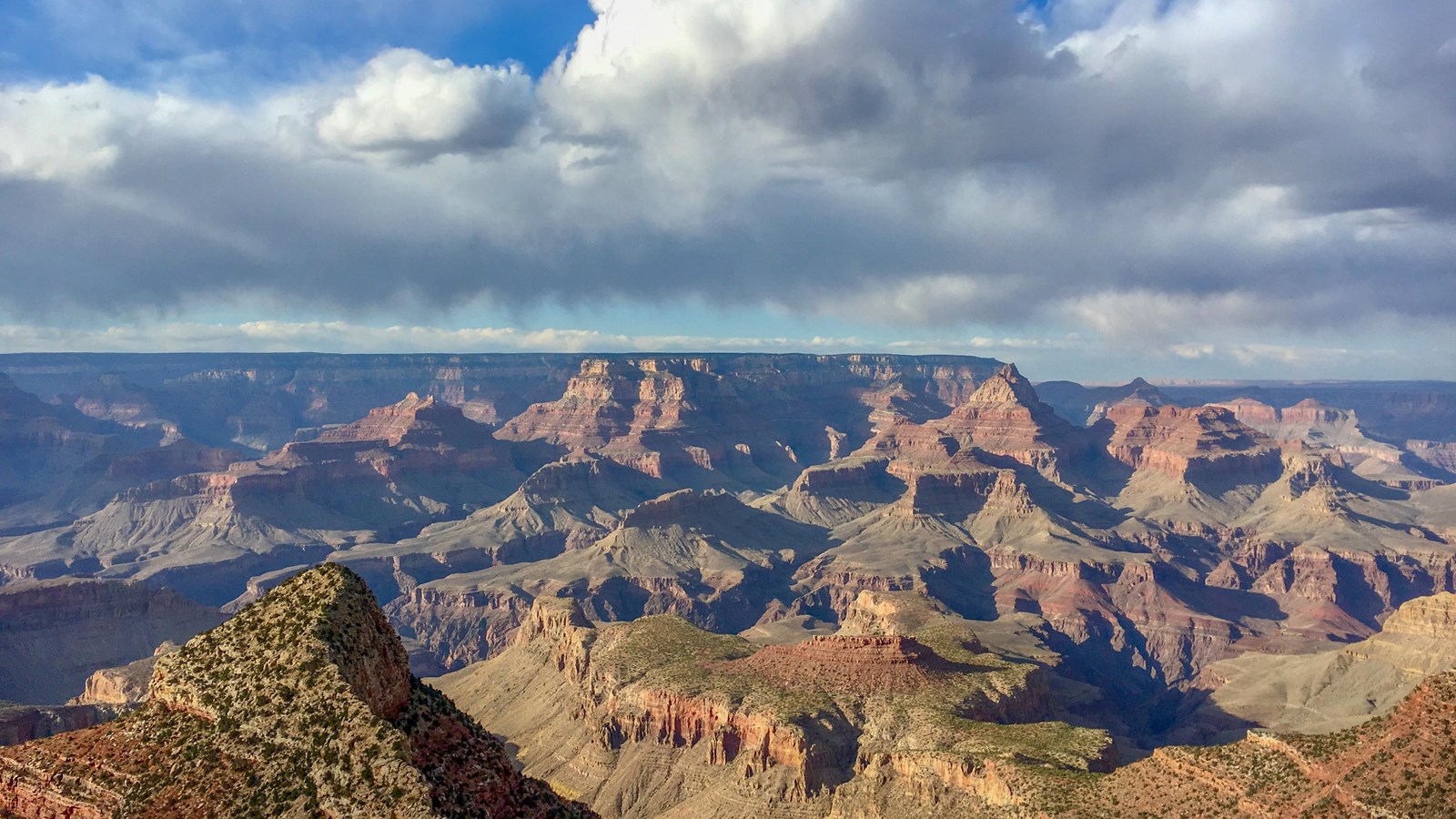A detailed landscape photograph showcases a rugged canyon, reminiscent of the Badlands or possibly the Grand Canyon, occupying about 60% of the lower portion of the image. The canyon's crevices and plateaus closer to the foreground are brighter tan with patches of green vegetation, while the distant sections transition to deeper, rusty reddish hues. Darker shadows cast across the canyon add depth to its rugged terrain. The upper 40% of the image is dominated by a brilliant blue sky, dotted with large, puffy cumulus clouds. These clouds have a striking white color with grayish-green undertones on their undersides, creating a dramatic contrast that highlights the expansive and raw beauty of the canyon below. Scattered patches of grass in the foreground and occasional green trees add additional texture and color to the scene.